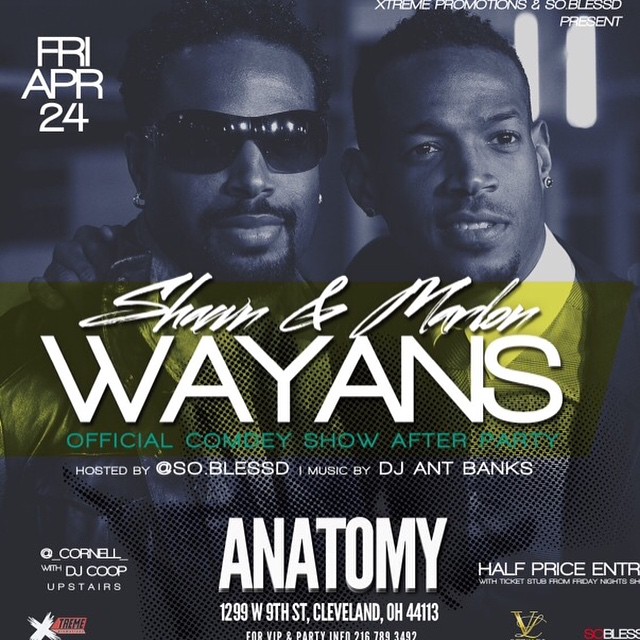This promotional poster advertises Sean and Marlon Wayans' official comedy show afterparty, hosted by So Blessed. The background is a black and white tinted blue photograph of the Wayans brothers, standing side by side. Sean, on the left, wears dark sunglasses, a black jacket with a scarf, and ear studs. Marlon, on the right, is facing the camera, with his right arm over Sean's shoulder. He sports a trimmed beard, short black hair, a black jacket, and a white shirt.

The poster features a gold horizontal banner with "Sean and Marlon" in bold white lettering, and underneath in larger white letters, "Wayans." Below their names, on a green background, it states "Official Comedy Show Afterparty."

In the upper left corner, the date "Friday, April 24th" is displayed in white lettering. The upper right corner reads "Extreme Promotions and So Blessed Present." The bottom center highlights "Anatomy" in big white letters on a dark background, along with the address "1299 West 9th Street, Cleveland, Ohio 44113."

For VIP and party information, a contact number is provided. The left side of the poster mentions "Cornell with DJ Coop upstairs," while the right side notes "Half Price Entry" with a ticket stub. At the very bottom, there's an "X" and a small banner that says "Extreme." In the lower right corner, a gold "V" with a "C" behind it, and text that reads "Bless" are visible.